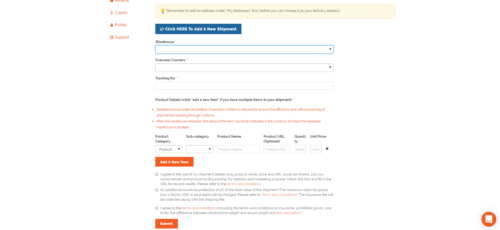The image showcases a comprehensive, web-based form designed for information input. At the top of the form, a yellow text box with black text provides initial instructions. Directly beneath this, a prominent blue bar functions as a clickable button for accessing further information. The form itself consists of several sections: first, a vertical stack of three text boxes designated for user inputs, followed by an orange text section imparting additional instructions. Below these instructions, more text boxes appear, each labeled with black headers for clarity. Toward the lower part of the form, a striking red button with white text offers another interactive element. Additional detailed instructions are provided below this button. At the very bottom of the form, there is another button intended for saving all entered data. Notably, a circular icon featuring a computer screen is situated in the lower right corner, possibly indicating technical support or additional functionality. Finally, the upper left corner of the form includes four menu options, each presented in orange text, providing users with navigational choices. Overall, the image depicts an intricate online form designed for seamless data entry and user guidance.